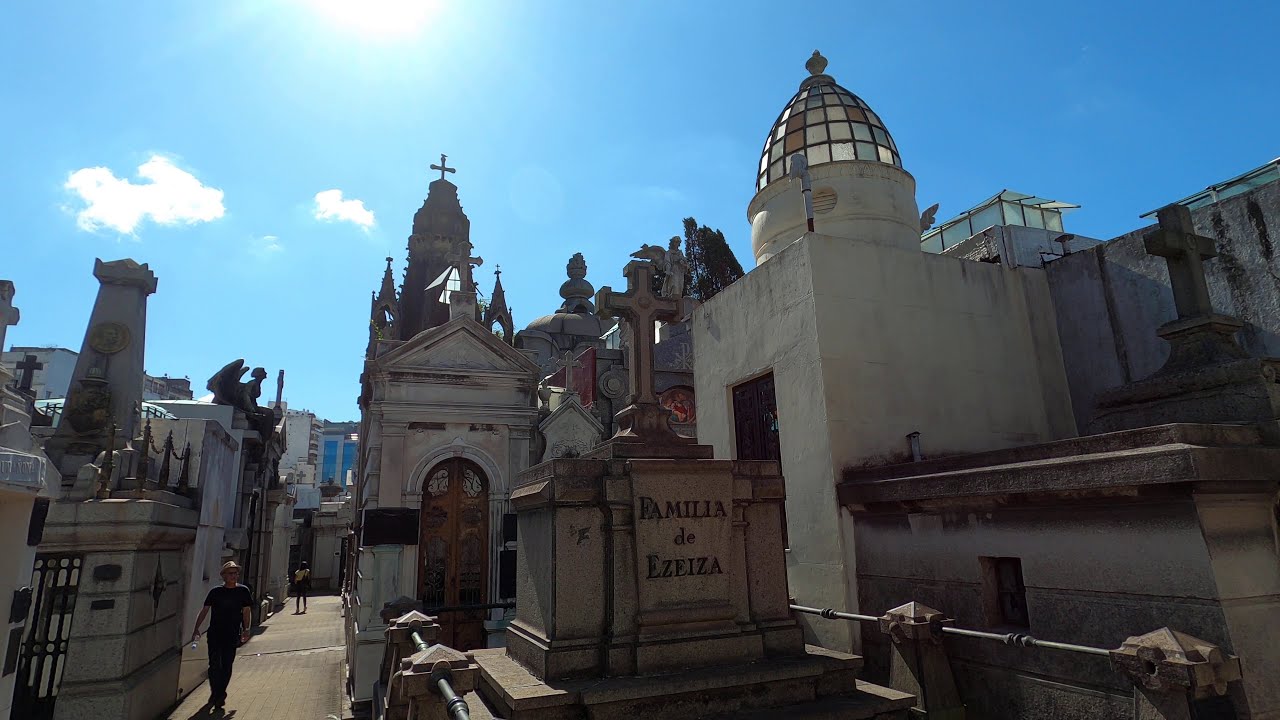This horizontally-aligned rectangular photograph captures a grand, ornate cemetery under a vast, clear blue sky punctuated by two feathery white clouds and a glimpse of the Sun at the top. Dominating the scene are numerous large, older stone buildings, resembling New Orleans or European-style mausoleums with intricate designs and crosses perched atop their domes. In the center of the image, there is a notable mausoleum with a stone cross and the inscription "Familia de Ezeiza." To its right stands a taller white stone structure with a dome adorned with stained glass and a crest. The left side features more stone buildings with an angel statue perched on one of them. Two people can be seen walking amidst this cemetery; a man dressed in all black—short-sleeved shirt and hat—walks towards the camera, while further away, a woman heads in the opposite direction. The scene is set on paths made of pavers, underscoring the cemetery's elaborate and antiquated atmosphere.